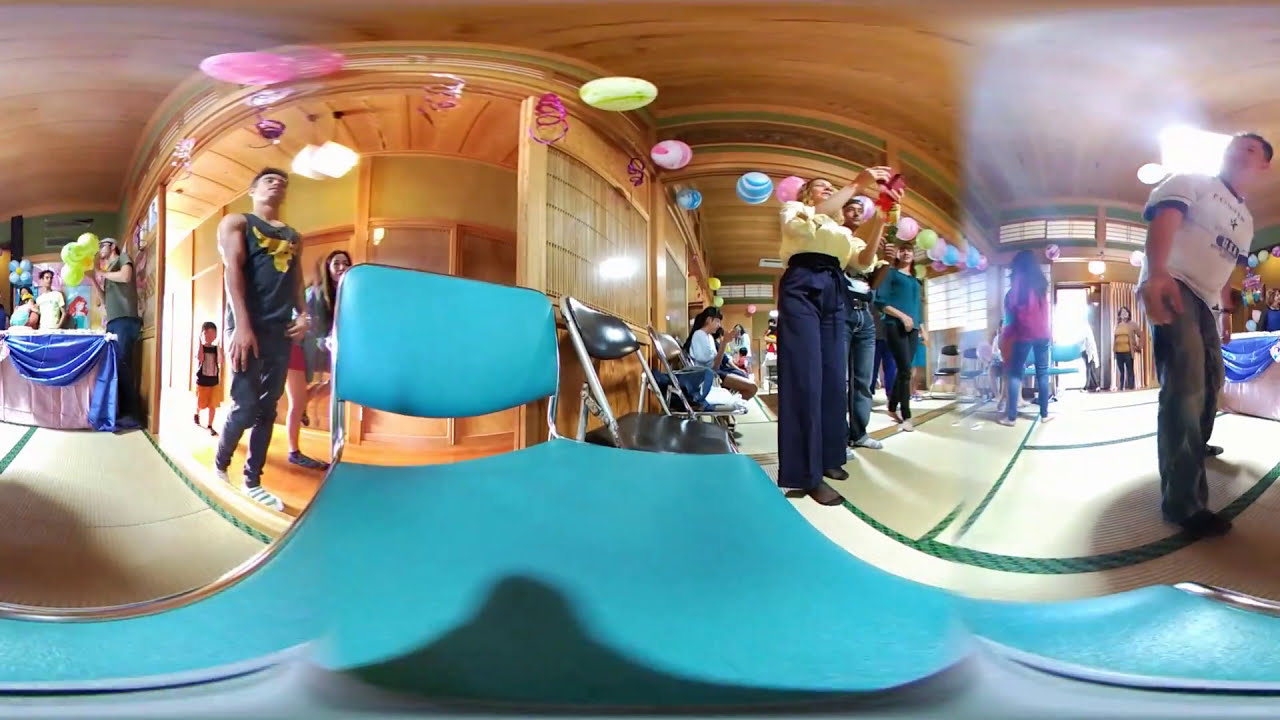The image depicts an indoor marketplace or party scene within a spacious area resembling a warehouse, characterized by wooden panel walls and ceiling. The space is bustling with around 20 shoppers and vendors, families with children, and individuals, some of whom are taking photos or looking at their phones while seated along the walls. The floor is a light green color with green edges. The left side of the image features what appears to be a wooden sauna and a table adorned with pink and blue tablecloths. Vibrant party decorations, including green and blue balloons and multicolored hanging spheres, suggest a festive atmosphere. Amidst the gathering, a man in a white shirt and dark pants stands on the right side, gazing upward. Despite the colorful decorations and various stalls, the scene conveys a somewhat muted energy, with many attendees appearing disinterested or bored.